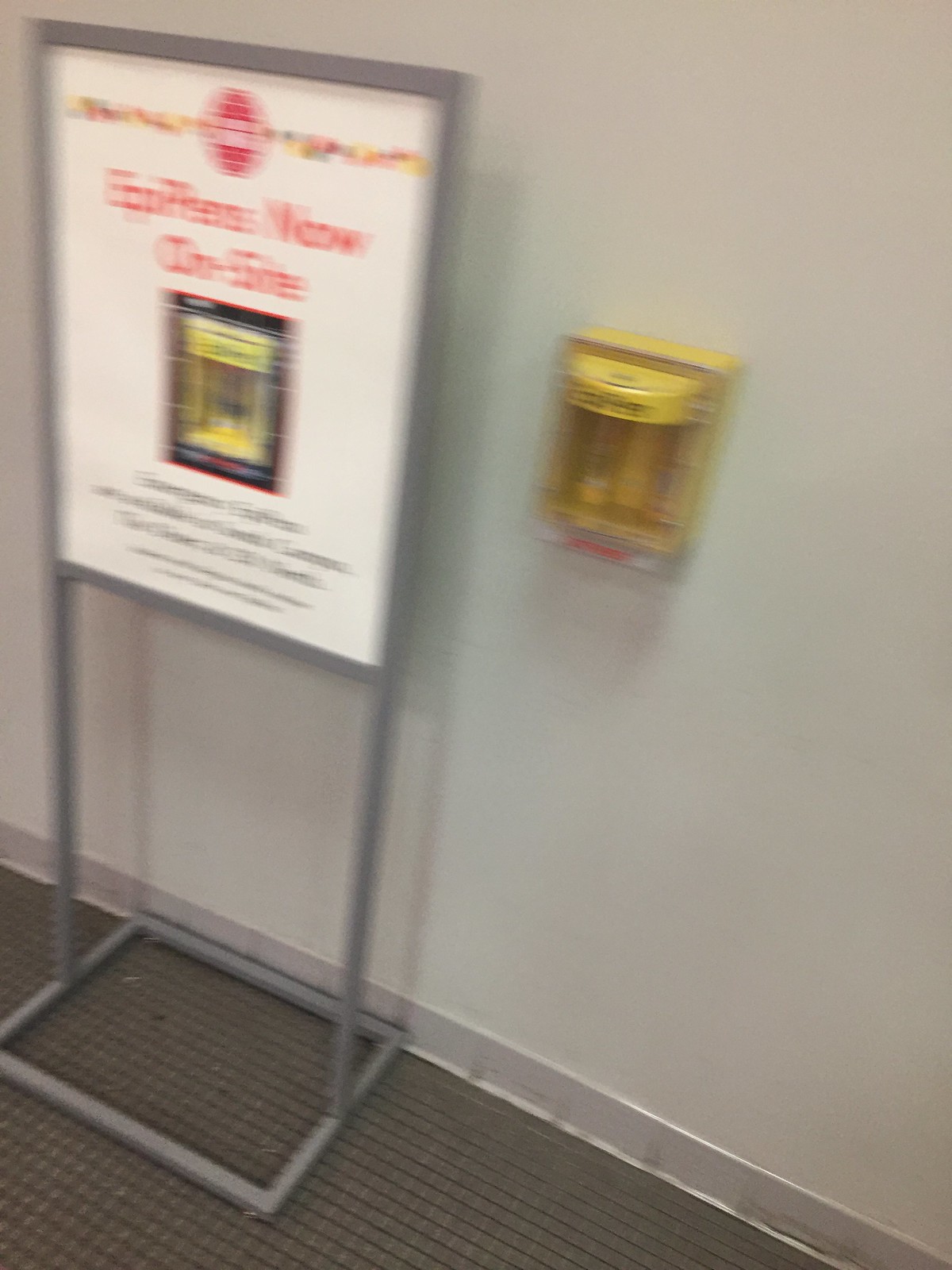The photograph depicts a blurry image of a black-framed, aluminum-style placard sign standing against a white wall. The sign has a hollow square base and vertical arms extending up to support a rectangular frame, within which lies a sheet of white paper or cardboard. The contents of the sign are mostly illegible due to the blurriness, but there appears to be red lettering at the top, a dark square image with a yellow background in the center, and some black writing underneath. To the right of the sign on the wall is a metallic fire pull device, commonly used to sound a fire alarm, although its details are also blurry and somewhat yellowish. Below, the white wall meets a gray molding that runs diagonally from center left to the bottom right corner. The floor is covered with an unattractive grayish-brown carpet. Though some text on the sign might suggest something like "EpiPens now on sale," this isn't clear, and it remains speculative.